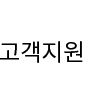The image is a minimalistic composition featuring a stark white background with four black characters, likely of East Asian origin, written in black ink. Each character is distinctly positioned from left to right. The first character resembles an L, comprised of two horizontal lines stacked with one at the top and one at the bottom, creating an almost opposite arrangement. The second character looks like a combination of a sideways V, an H, and an L at the bottom. The third is an upside-down V connected to a T on top, resembling a small tabletop with a vertical line to the right. The final character appears somewhat like a stick figure, with a circle at the top, a small L attached to the side, and a vertical line running upwards. Despite some viewers suggesting these could be Korean alphabet or kanji, the exact language of the characters remains uncertain.